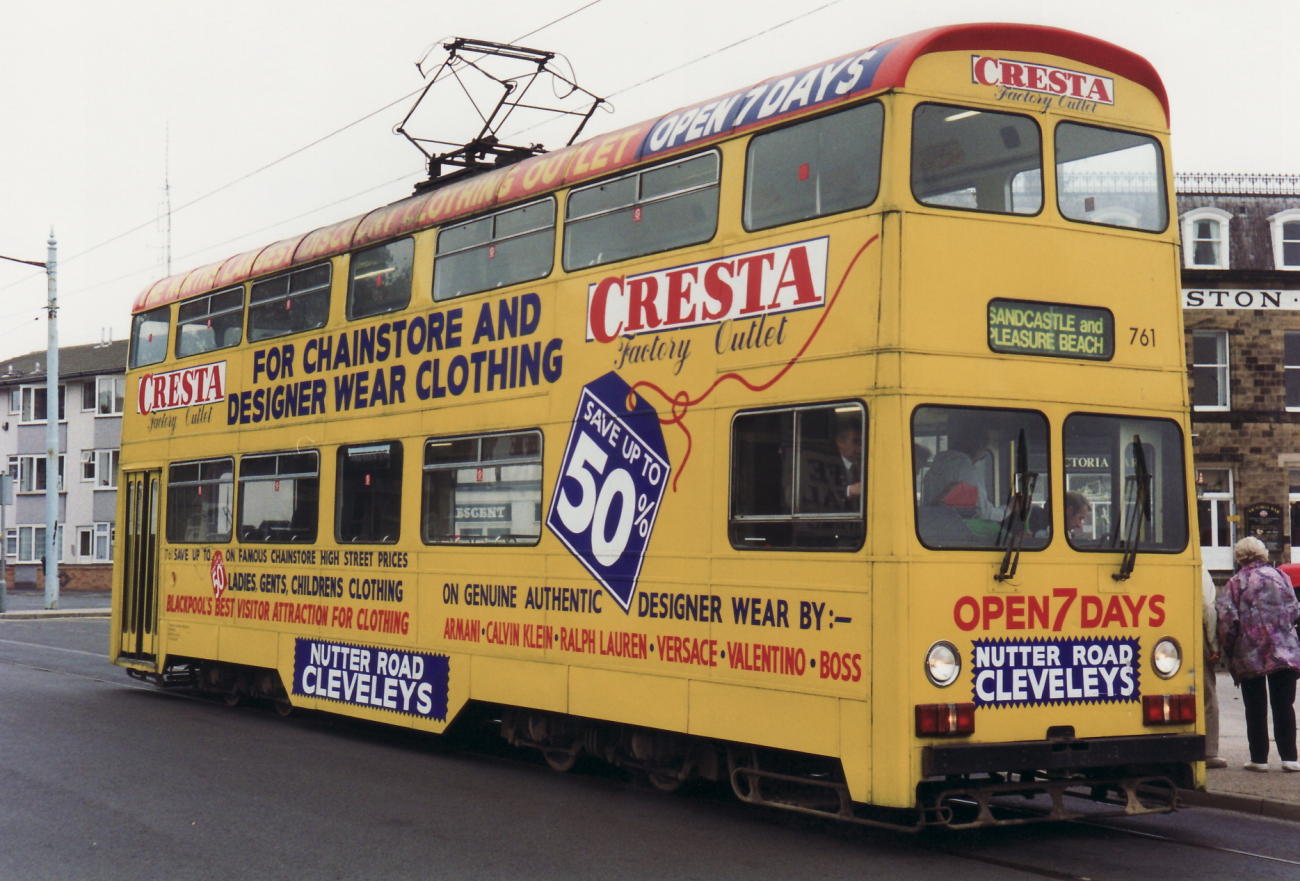The image depicts a bustling outdoor scene with a yellow double-decker bus prominently in the center. The bus is covered with a multitude of advertisements promoting the Cresta Factory Outlet, offering up to 50% off on genuine, authentic designer wear for ladies, gents, and children. The names of prestigious designers like Armani, Calvin Klein, Ralph Lauren, Versace, Valentino, and Boss are prominently displayed in red letters against a white background. At the top of the bus, a blue rectangle with white lettering announces "open seven days," alongside promotions for chain store and designer wear clothing. The bus sits on a road, with its upper section marked by two windows with windshield wipers, and a small sign reading "Sandcastle and Pleasure Beach." Above the scene, a gray sky and power lines stretch across the upper-left corner, while various buildings form the backdrop, adding depth to the urban environment.